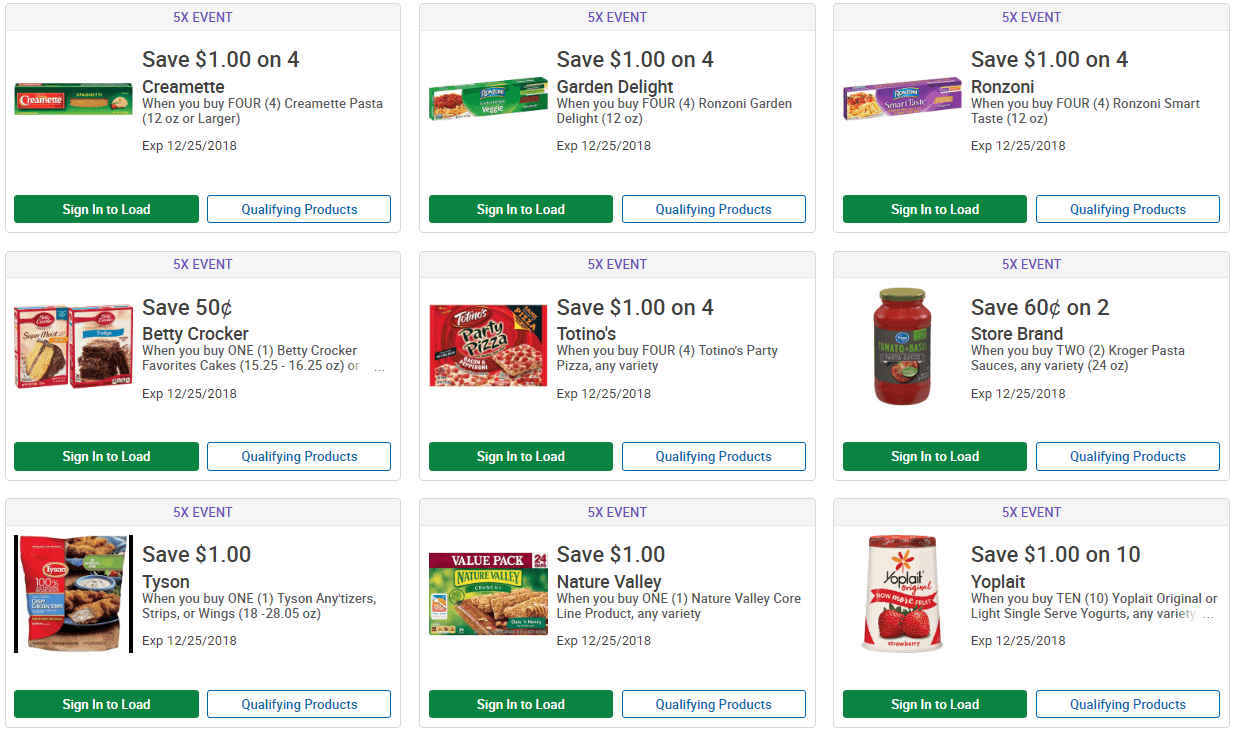This is a portrait-oriented screenshot showcasing search results for various products on a shopping website. The layout features a 3x3 grid with a total of nine products. Each product block is divided into distinct sections: 

- At the top, there is a gray header with a horizontal rectangular shape and blue font, indicating "5X event."
- Beneath this header is a white section displaying an image of the product, followed by a black header and a brief description.
- Below each product image, there is additional information such as savings and coupon details. To the left, within a green rectangular box, the text reads "Sign in to load," and to the right, a blue rectangle with a white background contains the phrase "Qualifying products" in blue font.

The nine products featured in the grid are as follows, along with their associated deals:

1. **Cremette** - Save $1 on four.
2. **Garden Delight** - Deal details not specified.
3. **Ranzoni** - Deal details not specified.
4. **Betty Crocker** - Deal details not specified.
5. **Totino's** - Deal details not specified.
6. **Store Brand** - Deal details not specified.
7. **Tyson** - Deal details not specified.
8. **Nature Valley** - Deal details not specified.
9. **Mule Plate** - Deal details not specified.

These products feature various coupons with savings ranging from $0.50 to $1. The image essentially highlights deals, discounts, and options for users to sign up and discover qualifying products for these promotions.